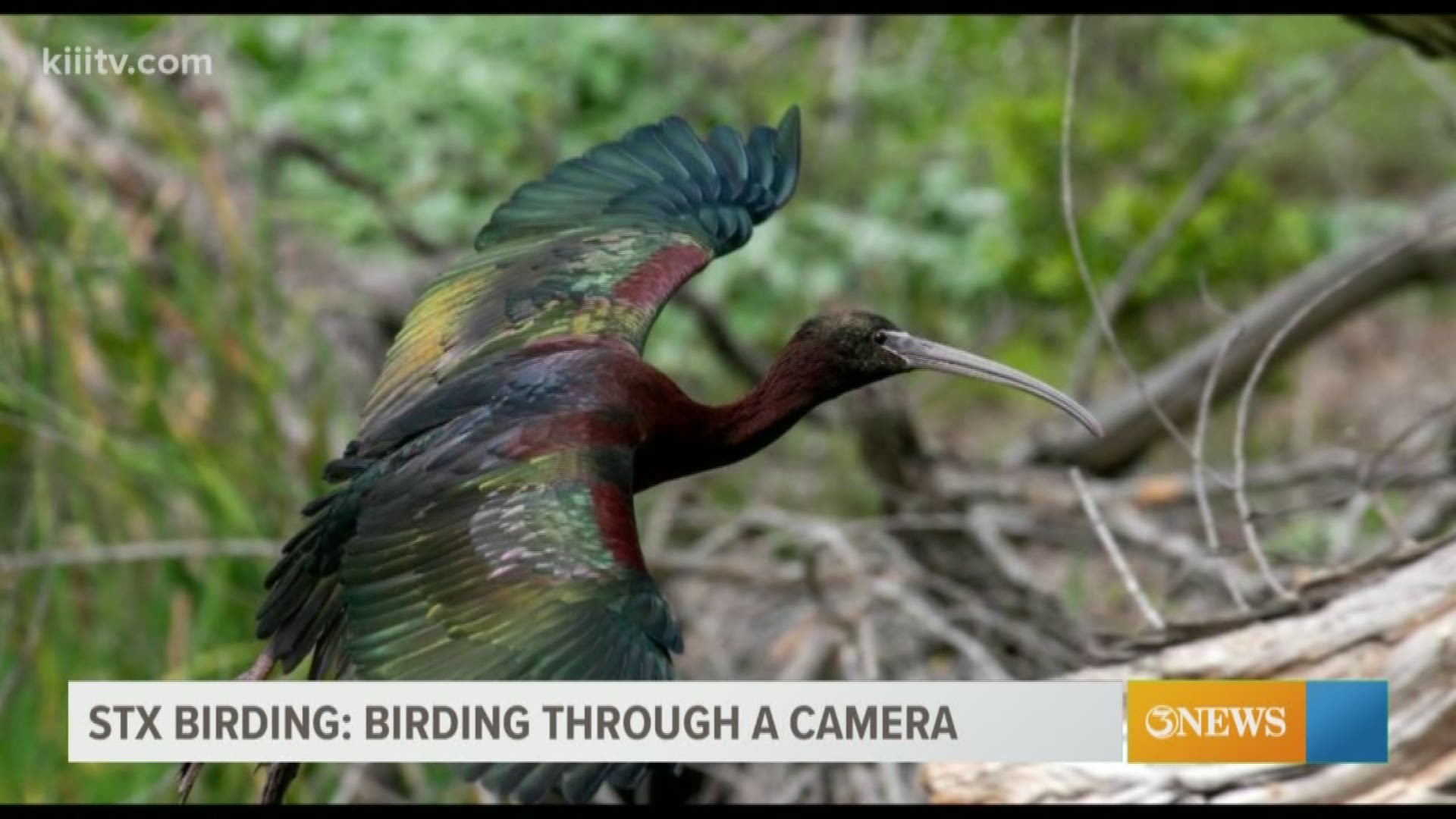This image, likely a screenshot from a news program, features a strikingly colorful bird in mid-flight against a blurred background of dark green foliage and scattered grey branches. Positioned in the center-left of the frame, the bird boasts a vivid reddish torso and a contrasting dark head, connected by a long, elegant neck. Its exceptionally long, thin grey beak curves gracefully to the right. The bird's expansive wings exhibit a dazzling, oil-like sheen with hues of green, blue, red, silver, and more, while its short tail fans out in dark blue. Thin black bars frame the top and bottom of the image. Overlaying the top left corner is a white watermark that reads kiiitv.com. Along the bottom is a white rectangle with grey text reading "STX birding, Birding through a camera," accompanied by an orange box with a white "3news" logo, right next to a blank blue box.